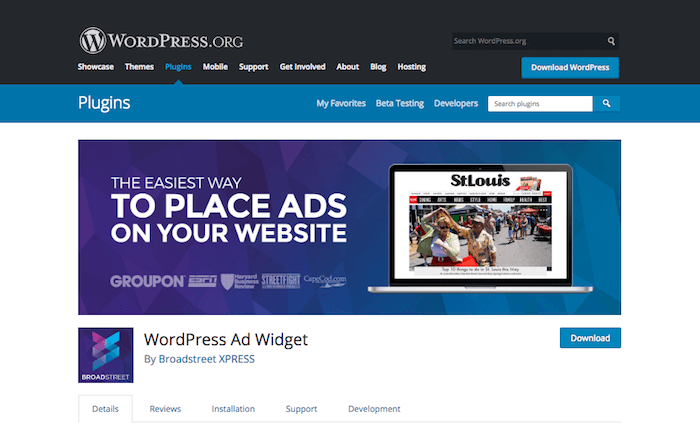The screenshot captures the homepage of the website WordPress.org. At the top, a black border displays the website name prominently. Just beneath this, there is a navigation menu with multiple clickable options: Showcase, Themes, Plugins, Mobile, Support, Get Involved, About, Blog, and Hosting. The Plugins option is highlighted, indicating it is the selected section, which is confirmed by a blue taskbar that extends below, featuring further options such as My Favorites, Beta Testing, Developers, and a search bar to find plugins. To the right, a noticeable blue button labeled "Download WordPress" offers a direct download option. Above, a subtly designed search bar with white text against a black background invites users to "Search WordPress.org." Dominating the lower section of the page, there is an illustrative box displaying a laptop screen showing what appears to be a website for St. Louis. Accompanying the image, a textual element to the left describes, "The easiest way to place ads on your website."